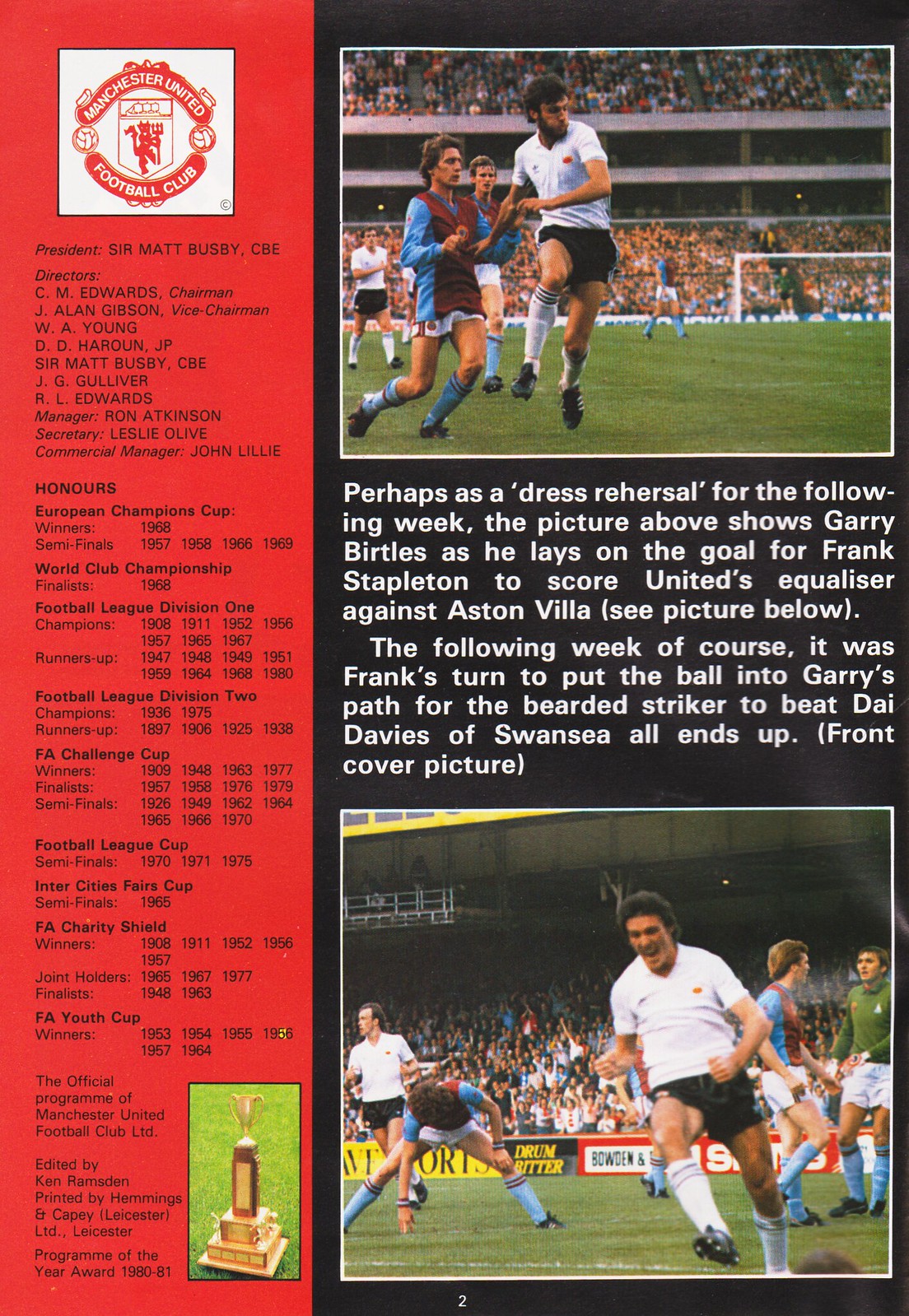This is an image of a detailed pamphlet from a Manchester United Football Club soccer program, presented in portrait format. The left side of the pamphlet is predominantly red and features the Manchester United emblem at the top, followed by a masthead listing the president, directors, managers, secretary, and commercial manager. Below, there are sections detailing the club's honors, championship years, and statistical history. 

The right side has a black background and is split into two parts by soccer player's photographs, one at the top and the other at the bottom. Both photos span the entire width of the black section, and in between them is white text. The text narrates a sequence of events describing a goal setup by Gary Birtles for Frank Stapleton's equalizer against Aston Villa, followed by a reverse scenario the subsequent week. The pamphlet's description emphasizes player interactions leading to goals, situating these moments as dress rehearsals for upcoming matches. The combination of red and black colors, along with detailed annotations and historical accolades, encapsulates the rich legacy and ongoing fervor of Manchester United Football Club.